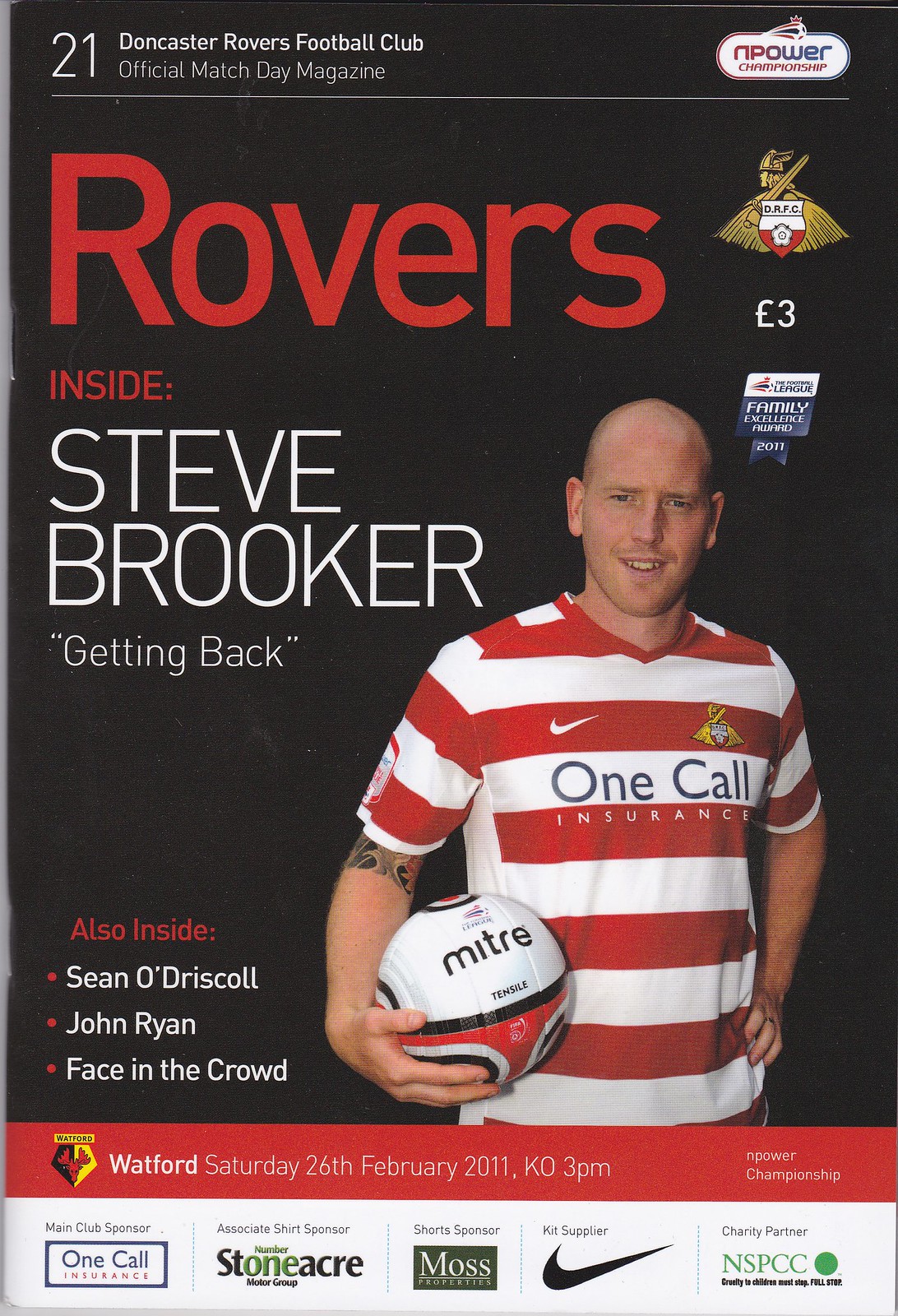### Detailed Caption

The cover page features a young, nearly bald Caucasian man with a receding hairline and blue eyes, smiling slightly to reveal his front row of teeth. He is standing at the center, wearing a red and white striped t-shirt with a Nike logo on one side and the words "One Call" in blue text, followed by "Insurance" in white text below. He is holding a volleyball close to his chest with one hand, while his other hand rests on his hip, revealing a tattoo just under the sleeve on his left arm.

Above him, in large text, it reads "21 Dorchester Rovers Football Club Official Match Team Magazine." There is an emblem on the right side that says "Empower Championship." The word "Rovers" is prominently displayed in large red letters. Below that, it states "Inside: Steve Brooker getting back." Further down the cover, it says, "Also inside: Sean O'Driscoll, John Ryan, face of the crowd." The bottom section of the cover features a red bar indicating "Waterford, Saturday, 26 February 2011, KO 3 PM, Empower Championship," followed by five advertisements in white for companies including One Call Insurance, Stoneacre, Moss, Nike, and NSPCC. The overall background of the cover is a very dark black.